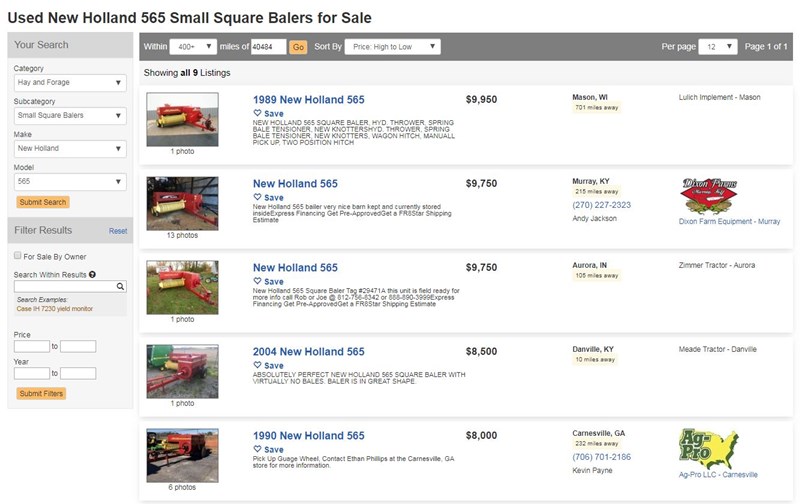Screenshot of a Classified Listing for Used New Holland 565 Small Square Balers:

At the top of the screenshot, there is a heading that reads "Used New Holland 565 Small Square Balers for Sale." To the left side, a vertical menu allows users to refine their search with various categories and filters, including options like 'Your Search,' 'Category: Hay and Forage,' 'Subcategory: Small Square Balers,' 'Make: New Holland,' 'Model: 565,' and buttons for 'Submit Search,' 'Filter Results,' and 'Reset.' Additional filters include preferences for 'For Sale by Owner,' 'Search within Results,' 'Search Examples,' 'K7230 Yield Monitor,' alongside input fields for 'Price: [blank to blank]' and 'Year: [blank to blank].'

A rectangular gray banner at the top allows sorting options within a 400+ miles radius of ZIP code 40484. It also includes sorting choices such as 'Sort by Price High to Low,' with pagination set to display 12 listings per page, currently on page 101.

The listing features multiple photographs and descriptions of available balers:

1. **1989 New Holland 565** - Priced at $9,950, located in Mason, WI (701 miles away), listed by Lufic Implement Mason.
   
   ![Red Baler Image]

2. **New Holland 565** - Priced at $9,750, located in Murray, KY (250 miles away). The listing highlights the condition as "Very nice, barn kept, and currently stored inside." The options mention "Express financing available" with the ability to "Get pre-approved" and "Get a free star shipping estimate". For more details, contact Andy Jackson at Dixon Farm Equipment, phone number 270-227-2323.
   
   ![Red Baler Image]

3. **New Holland 565** - Another unit priced at $9,750, located in Aurora, IN (105 miles away), listed by Zimmer Tractor, Aurora.
   
   ![Red Baler Image]

4. **2004 New Holland 565** - Listed at $8,500, described as "Absolutely perfect New Holland 565 square baler with virtually no bales, in great shape." Located in Danville, KY (10 miles away), and listed by Mead Tractor, Danville.
   
   ![Red Baler Image]

5. **1990 New Holland 565** - Priced at $8,000 and described as having a "Pick-up gauge wheel." For further information, contact Ethan Phillips at the Carnesville Georgia store, 706-701-2186. Location: Carnesville, GA (232 miles away). The listing is managed by Kevin Payne from Agpro LLC, Carnesville.
   
   ![Red Baler Image]

Each baler is depicted in a photograph, predominantly showcasing in red, and features specific details about the model, condition, price, and contact information for inquiries.